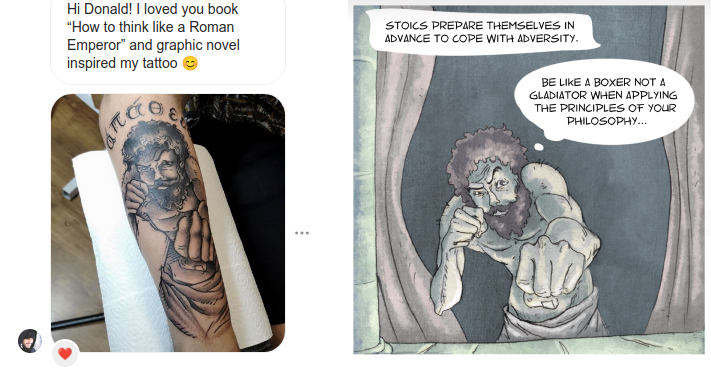The image consists of two parts: the left side shows a photo of a man's forearm tattoo, while the right side depicts the source of inspiration—an illustrated scene from a graphic novel. The tattoo spans from just below the elbow to the wrist, featuring a realistic black-and-white image of a bearded man with shaggy hair. The man is shirtless, wearing a towel around his waist, and positioned as if in a fighting stance, with his left fist extended and his right fist near his chin. The tattoo is displayed on a white cloth on top of a brown table. Above the tattoo in a text bubble, it reads: "Hi Donald, I loved your book How to Think Like a Roman Emperor and graphic novel inspired my tattoo."

On the right side, the graphic novel scene mirrors the tattoo, depicting the same bearded man in a fighting stance. Above the illustration, there’s a thought bubble stating: "Prepare themselves in advance to cope with adversity," and another thought bubble to the right of the character's head that reads: "Be like a boxer, not a gladiator when applying the principles of your philosophy."